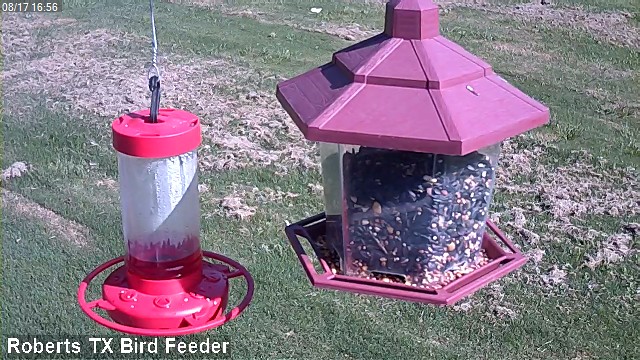This horizontal rectangular photograph captures an outdoor scene under a sunny sky, evident from the well-lit background of short grass interspersed with patches of dead grass. The image is taken from an elevated height of approximately 50 feet, looking down at a slight angle towards two bird feeders.

On the left, there is a hummingbird feeder featuring a circular red top, a clear cylindrical middle, and a circular red base with a ring designed for feeding birds. On the right, a slightly larger bird feeder stands with a burgundy red, hexagonal top, a clear central tube filled predominantly with black sunflower seeds, interspersed with yellow and white seeds, and a maroon-colored hexagonal base with ledges for birds to perch on.

In the upper left corner of the image, there is a timestamp displaying "08/17, 16:56" in white text with a black, slightly transparent rectangular background. In the lower left corner, similar text indicates "Roberts TX Bird Feeder."